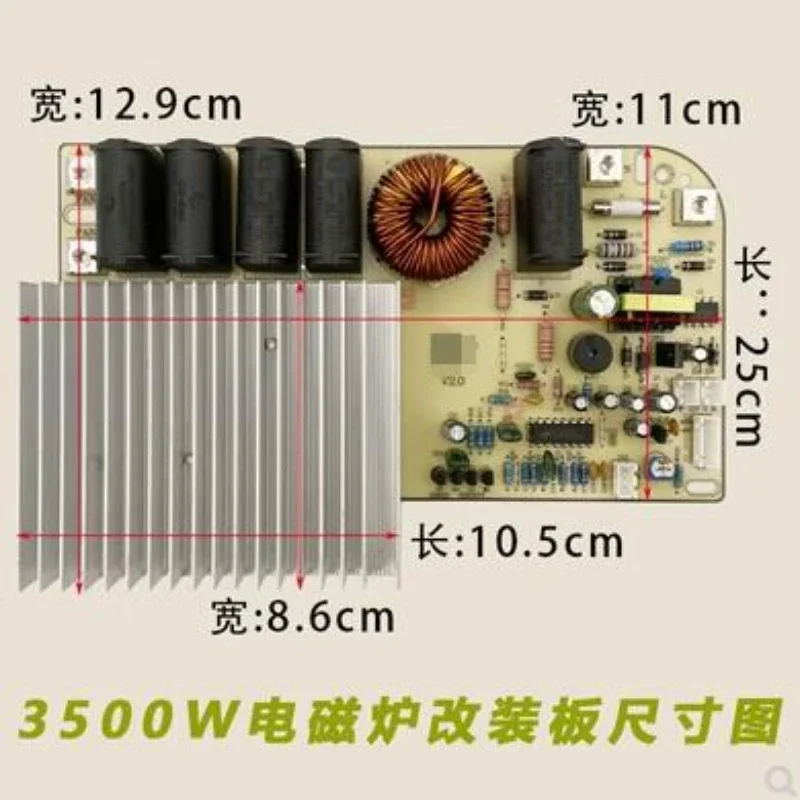This is a detailed photograph of an electrical equipment piece, likely a computer motherboard, set against a tan background. The primary component is a light green rectangular board, with the upper right-hand corner slightly rounded. Prominently featured are five black cylindrical tubes at the upper left-hand corner, with four of them aligned vertically and reaching halfway down the board. Adjacent to these cylinders is a copper wire wound into a donut-like shape, flanked by another similar cylindrical tube. The right side of the board is crowded with various circuit breakers and components of differing shapes and sizes, including squares and circles, arranged in rows.

On the bottom left, beneath the four black cylinders, hangs a metal sheet resembling an accordion due to its vertical lines. This sheet extends beyond the lower and left edges of the motherboard. Red arrows and thin lines, drawn over the entire image, form a grid pattern and indicate measurements, highlighting specific dimensions in centimeters alongside Chinese characters. Dimensions specified are 12.9 cm on the left side, 11 cm in the upper right corner, 25 cm on the right side, 10.5 cm on the bottom right, and 8.6 cm beneath the metal plate. The bottom of the photograph features the text "3500W" in an olive green color, accompanied by additional Asian characters.